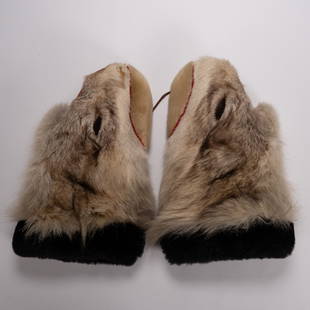This up-close photograph depicts a pair of intricately detailed, ankle-high fur shoes, positioned against a stark white background, likely in a museum setting. The shoes feature a unique combination of materials and colors: the toe area is covered in dense black fur, while the body of the shoe is enveloped in a mix of fluffy brown and tan fur, potentially sourced from rabbit. The wide, rectangular-shaped toe boxes stand out prominently. Towards the heel, there is a small slit designed for foot insertion. The heels themselves appear to be crafted from suede or animal skin. Notably, the shoes also feature black elastic bands near the top, suggesting a design element reminiscent of animal heads with pointed ears, giving them an almost mitten-like appearance. These elastic bands and the surrounding cream-colored background contribute to the overall visual appeal of the exhibit.